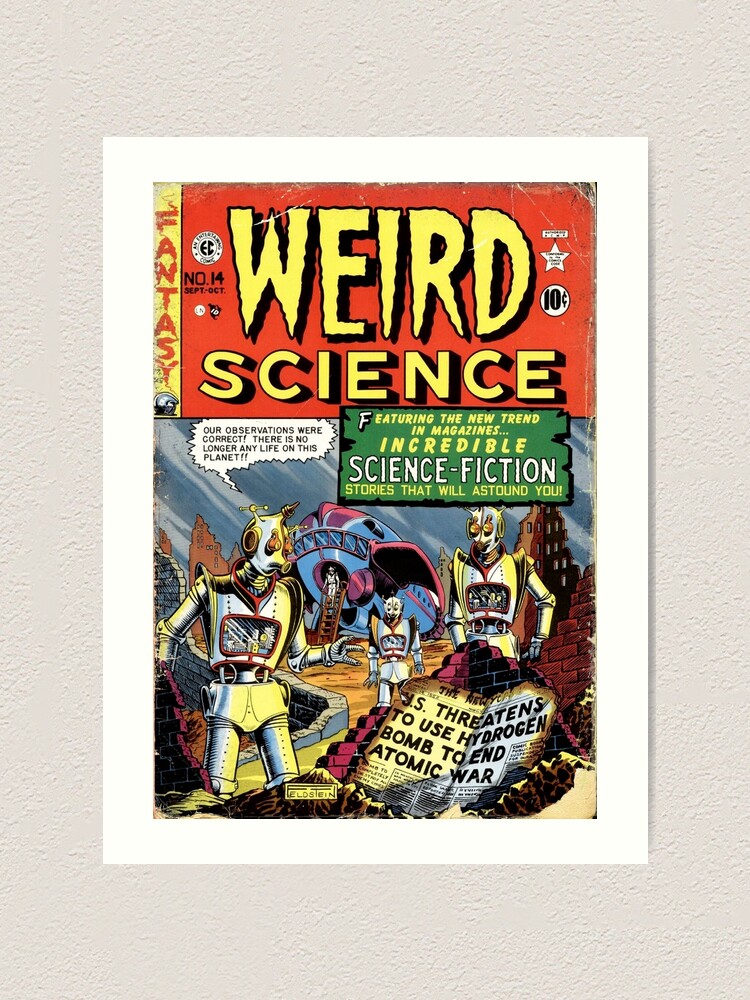The image is the front cover of a vintage comic book titled ‘Weird Science.’ The title is prominently displayed in large, bright yellow capitalized letters against a red background. To the left of the title, the word ‘Fantasy’ is written. Below the title, within a green box, it states, "Featuring the new trend in magazines, incredible science fiction stories that will astound you." The book is issue number 14, priced at 10 cents, dated September and October.

The cover art depicts a colorful and busy scene. Futuristic robotic or armored figures, possibly aliens or humans in strange outfits resembling underwater masks, are seen descending from a blue and purple spaceship onto a rocky planet surface via a brown ladder. To the upper left, a comic bubble reads, "Our observations were correct. There is no longer any life on this planet." In the foreground, a burnt-looking newspaper headline declares, "U.S. threatens to use hydrogen bomb to end atomic war," adding a sense of urgency and historical context to the scene. The overall illustration is highly detailed, capturing the essence of mid-20th century science fiction.